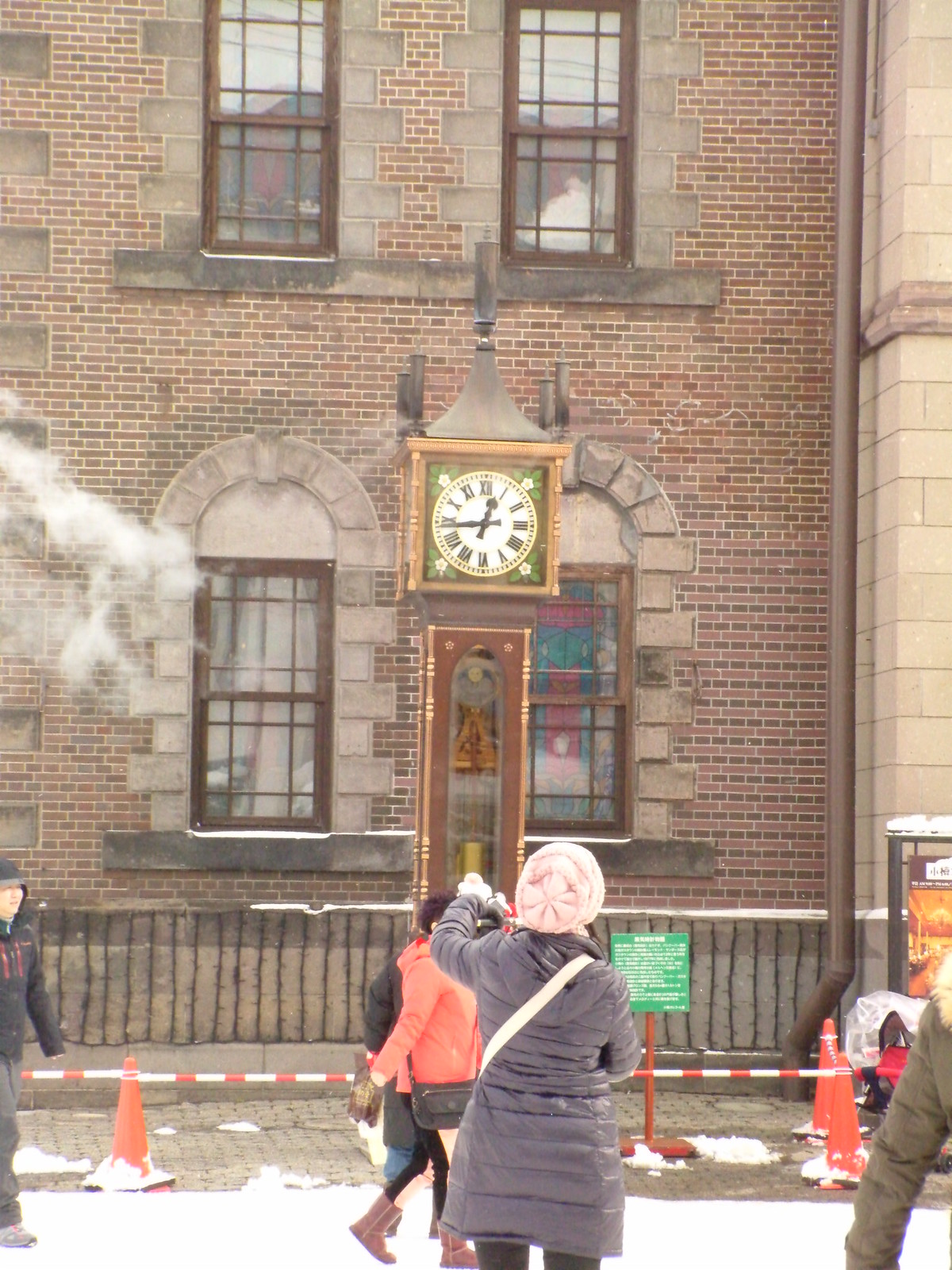A detailed photograph showcasing a serene city street in an old European town. In the background stands a striking building constructed from red and brown bricks, adorned with intricate cathedral-style stonework enveloping the square wooden, paned windows. The centerpiece of the scene is an imposing outdoor clock resembling a grandfather clock but on a much larger scale. Its clock face is white set against a green backdrop, and the ornate clockworks, including the pendulum and clock weights, are highlighted in a golden brown color, with gilded edges adding a touch of opulence.

On the street in front of the clock, red and white striped traffic cones and barrier tapes section off areas, perhaps for maintenance or an event. A small, square sign with a green face and fine print, likely providing details or history about the clock, is positioned nearby. People clad in winter attire—coats, hats, and boots—populate the street, suggesting a chilly season. Patches of snow dot the ground, completing the picturesque winter cityscape.